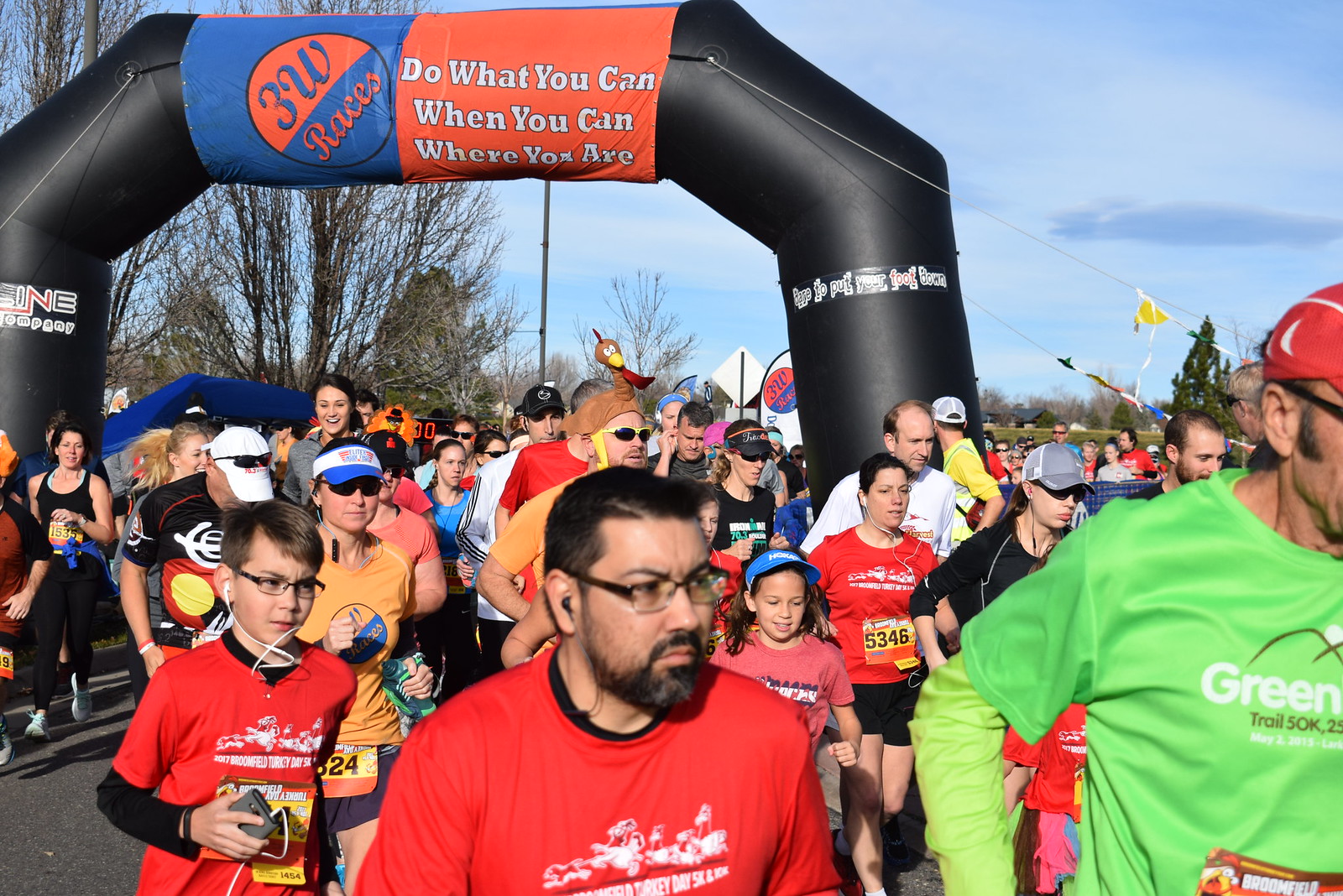In the image, we see the start of a running event, marked by an inflatable archway that reads "3W Races" on one side and "Do what you can, when you can, where you are" on the other. The archway, black on the sides and connected to the ground with strings, stands prominently at the starting line. Participants of various ages are running together in a dense group, slowly making their way forward, each wearing numbered bibs such as 5, 3, 4, and 6 pinned to their jerseys. 

Right in front of us is a gentleman in a green jersey and another runner in the middle wearing a red T-shirt and glasses. Among the crowd, many runners are outfitted in baseball hats and sunglasses. We notice one young runner with earpods and a device playing music. The scene is set against a backdrop of a blue, slightly hazy sky, with sparse trees and a wide open area, giving the impression that the race is taking off from a park or a similar venue.